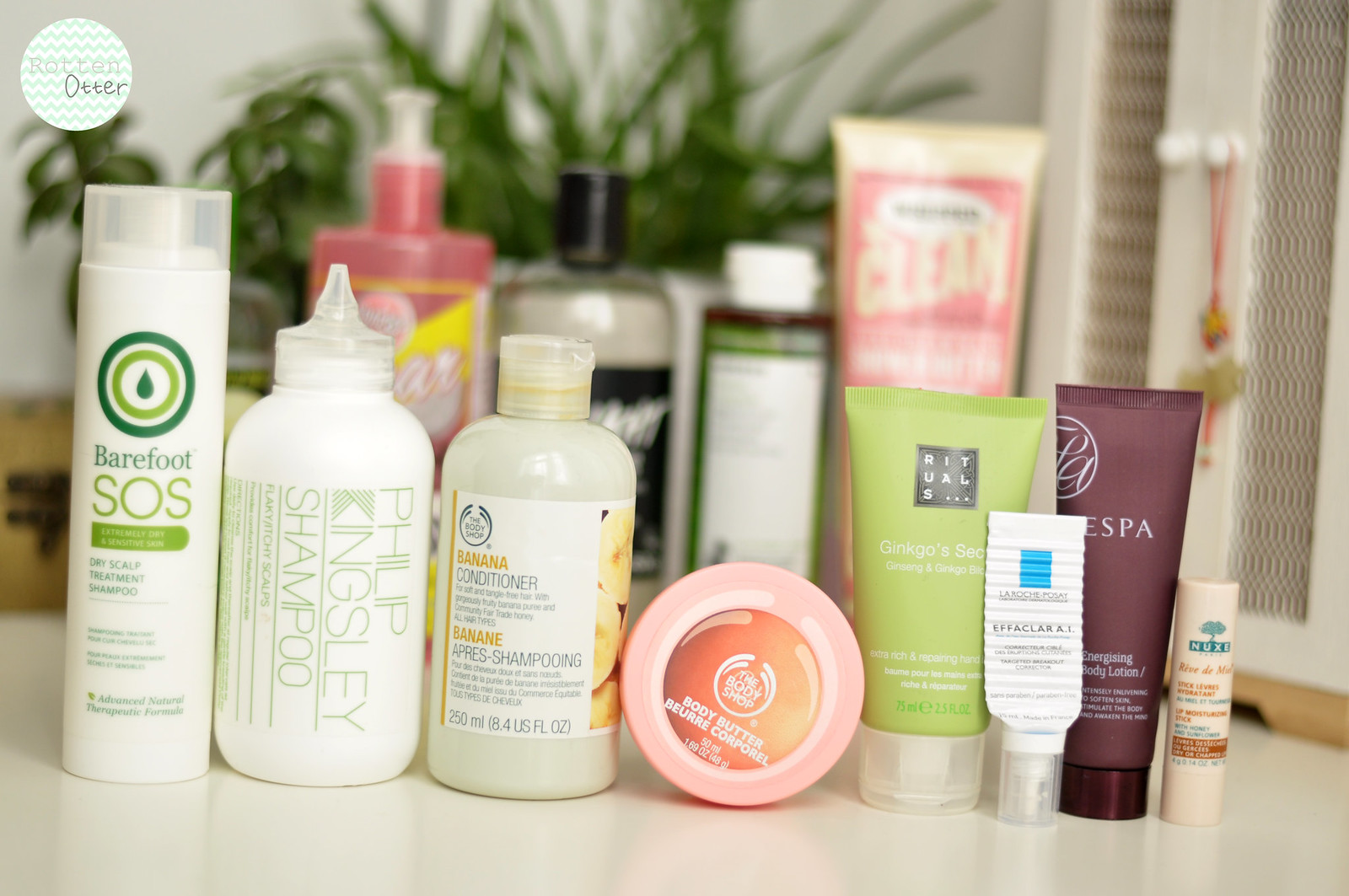This image depicts a collection of beauty products meticulously arranged on what appears to be a bathroom sink unit, illuminated by soft lighting that highlights each item. The surface, likely serving as a bathroom worktop, holds an impressive assortment of high-quality beauty and personal care products, possibly curated for resale on platforms like eBay, Vinted, or Gumtree. In the background, there is an eye-catching, Ikari-style wardrobe made of a combination of crisp white-painted wood or white vinyl wood with a base of rustic pine. The wardrobe's doors are adorned with dense, corrugated plastic panels that obscure any view of the interior, and they feature sleek, white doorknobs. A delicate touch is added by a miniature ballerina figurine in a tutu, elegantly suspended from one of the door handles, adding a whimsical charm to the setting.

On the bathroom sink unit, the beauty products are neatly laid out, showcasing a variety of premium brands and treatments. These include Barefoot SOS skincare, Philip Kingsley shampoo, and The Body Shop's nourishing Banana Conditioner. Additional items include a tub of The Body Shop's renowned body butter, a selection of luxurious Rituals products, and quality offerings from ESPA. This curated collection emphasizes both high-end beauty and self-care, appealing to a discerning audience keen on premium personal care items.